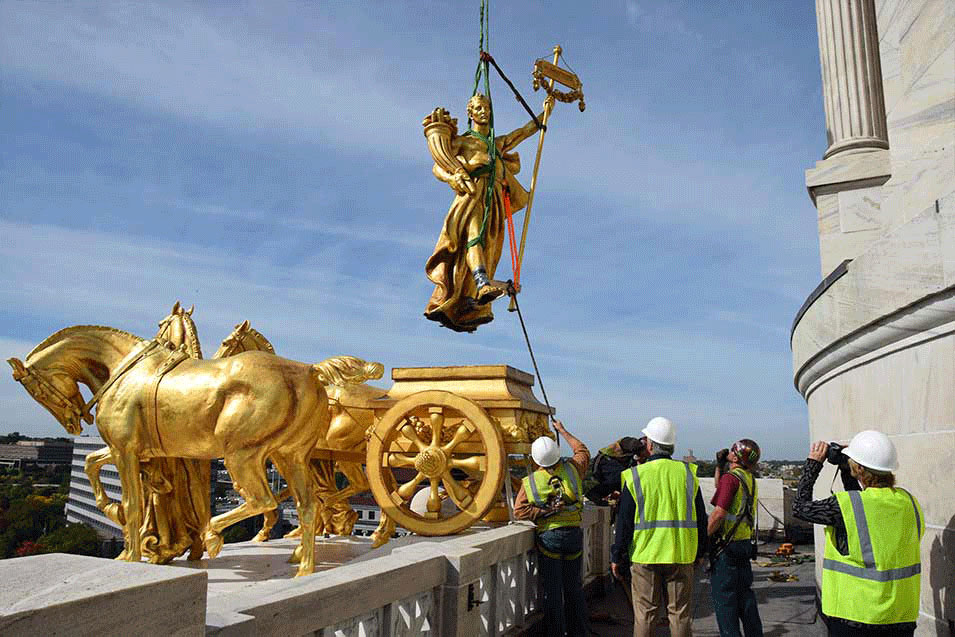In this detailed image, construction workers are meticulously positioning a golden statue onto a white ledge on a balcony. The statue, portraying a goddess-like figure in a flowing dress, is being carefully lowered by green and orange ropes. The figure majestically holds a cornucopia in one hand and a gold scepter with a banner in the other. On the balcony below, an already-installed golden base features intricate sculptures of horses pulling a chariot. The workers, clad in high-visibility lime green safety vests with reflective silver stripes and white and yellow hard hats, are either managing the ropes or observing the delicate operation. The scene is set against a backdrop of a grand marble building with visible columns and a half-wall, and the sky is a serene blue adorned with thin, wispy clouds.